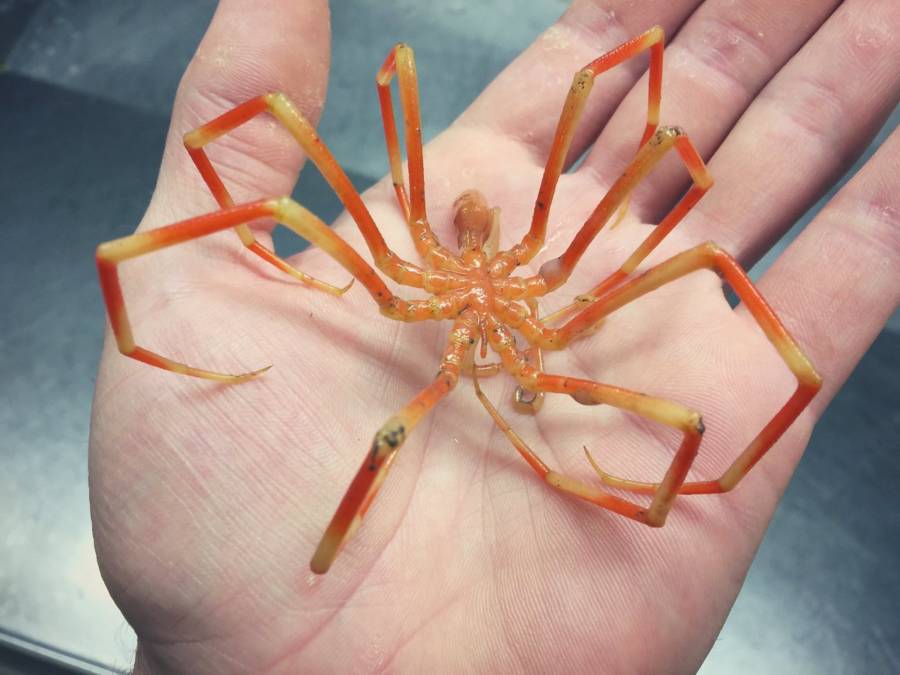The image showcases a large, eerie-looking spider, predominantly yellow and orange with thin, striped legs, and a flat, elongated body. The spider, with its eight spindly legs ending in talon-like points, is cradled in the palm of a person's hand, which appears dry and slightly peeling. The spider is positioned directly in the center of the photograph, slightly towards the top, and is highlighted against a grayish-blue background that suggests the hand is hovering over a table or metal surface. The detailed colors in the image include silver, gray, black, yellow, orange, and peach, and the scene could be set in either a home or a laboratory studying spiders.